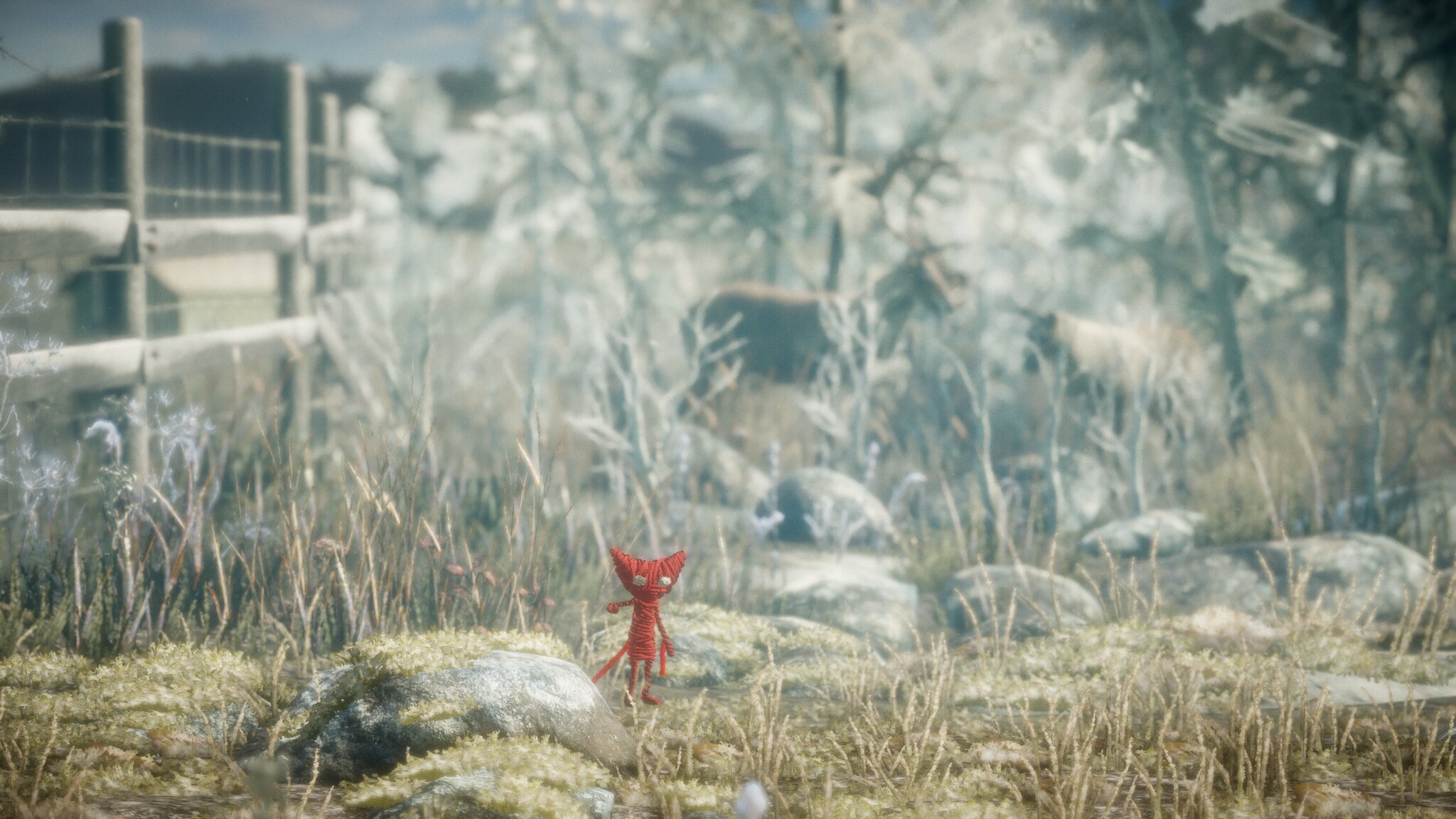In this detailed image, we encounter an illustrated scene that centers on a small, red, cat-like figure characterized by its upright stance, white eyes, and two prominent horns. The figure appears to be fashioned from yarn, with noticeable loose threads on its outstretched right arm and left hip. This endearing character stands amidst a diverse landscape of green rocks and both short and long grass. In the upper left, a green bridge arches gracefully, while a clear blue sky with scattered white clouds adds depth to the backdrop. To the right, gray-hued trees further frame the setting. The background also features a white flower and more dry weeds interspersed with blurred, large animals resembling horses, suggesting a tranquil farm or grassy field environment. A fence supported by concrete columns subtly lines the scene, enriching the picturesque and pastoral ambiance.